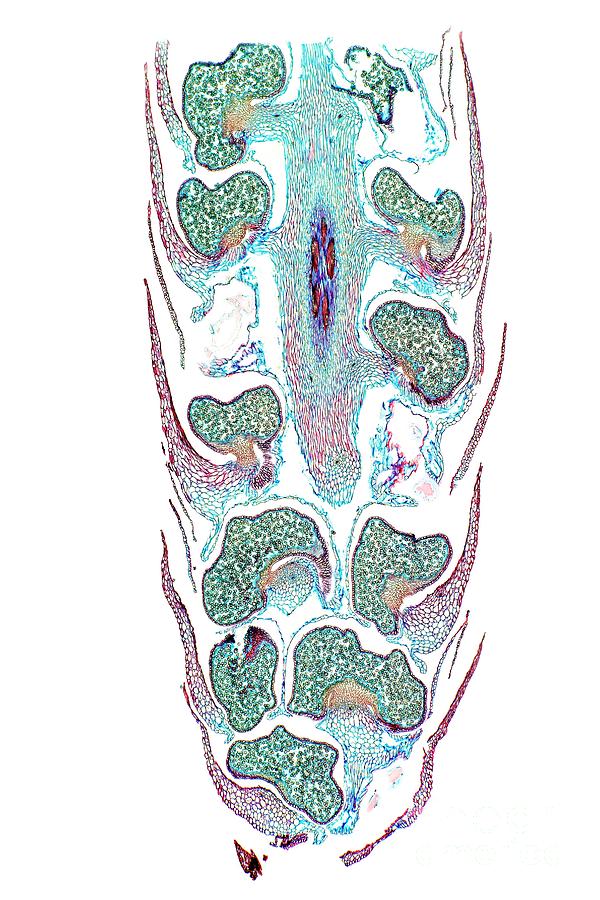The image is a detailed, vibrant depiction that could be of a cell as viewed under a microscope or a colorized cross-section, possibly from a CT or x-ray scan, presented in an artistic manner. The central focus of the image features a striking red and blue line bisecting the length of the piece, which might represent a central structure or axis within the cell. Surrounding this central line are various colorful blobs in hues of red, blue, green, and pink. The red blobs are notably spiky and form an outline around the more amorphous green blobs. At the center top, there is a prominent light green structure with a bright red core enveloped by a purple aura, which drips downward, blending into the surrounding colors. The bottom part of the image shows clusters of cells in light blue and green, with the green fading into the red that forms the cell’s boundary. The interstitial spaces are tinged with white or lighter shades, adding to the image’s layered complexity. This image, rich in color and detail, could serve as both a scientific illustration and an aesthetically pleasing art piece suitable for display.